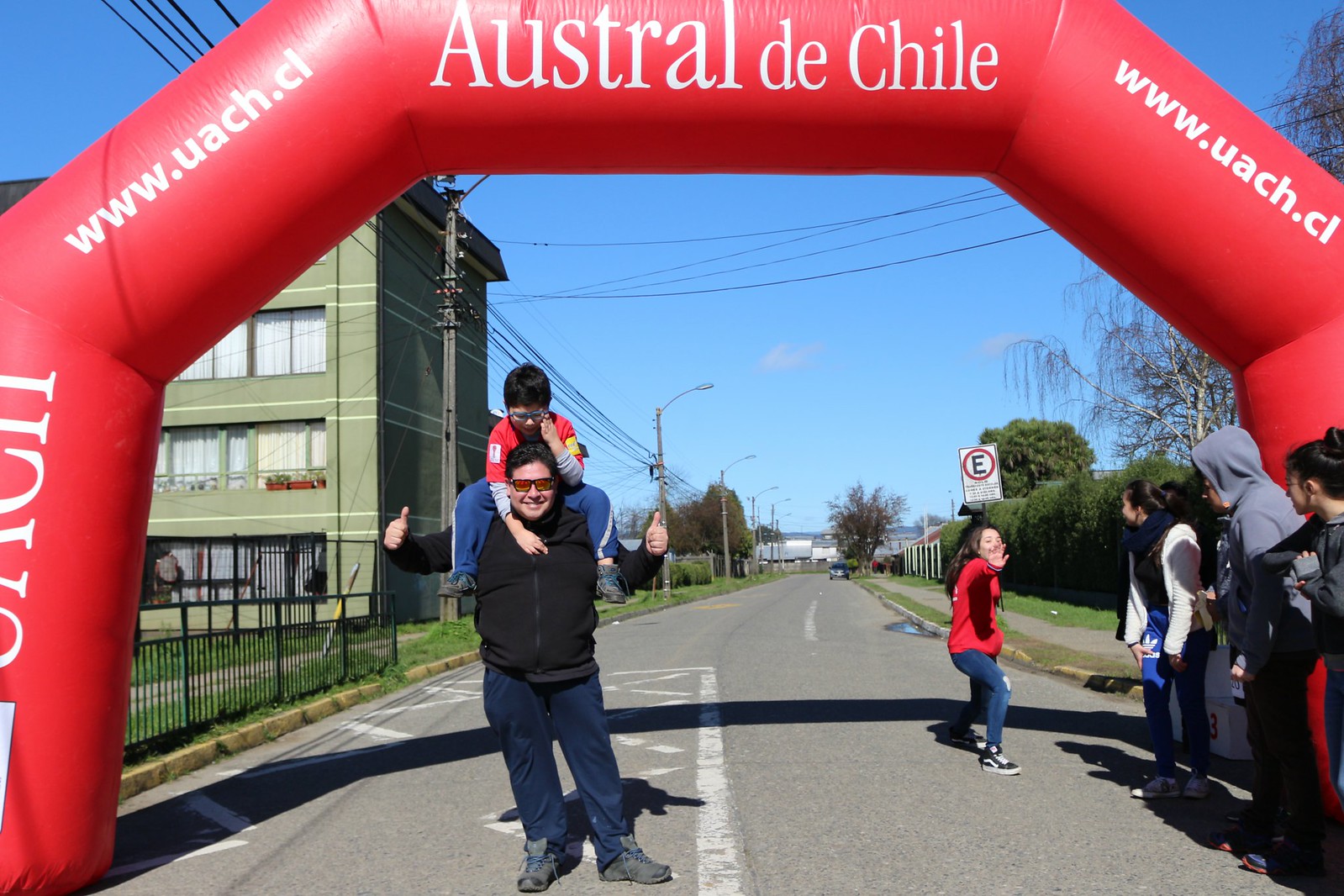The image captures the vibrant end of a race under a striking red inflatable arch that reads "Austral de Chile" at the top and "www.uach.cl" on the diagonal sides. Underneath the arch, a cheerful man, wearing reddish sunglasses, a black jacket, dark blue jeans, and gray shoes, stands with his arms stretched out, giving a double thumbs up. Seated on his shoulders is his young son, who also wears glasses, a red shirt over a bluish long-sleeve shirt, and dark blue pants. To the right, a crowd of spectators, including a woman with long brown hair and a red top, stands eagerly waiting. Behind them, the sky is a bright blue with a few scattered clouds and telephone wires. The left side of the scene features a green multi-storey building and a small pavement beyond grassy areas. A car is visible in the background, approaching the finish line, adding to the scene of excitement and anticipation.